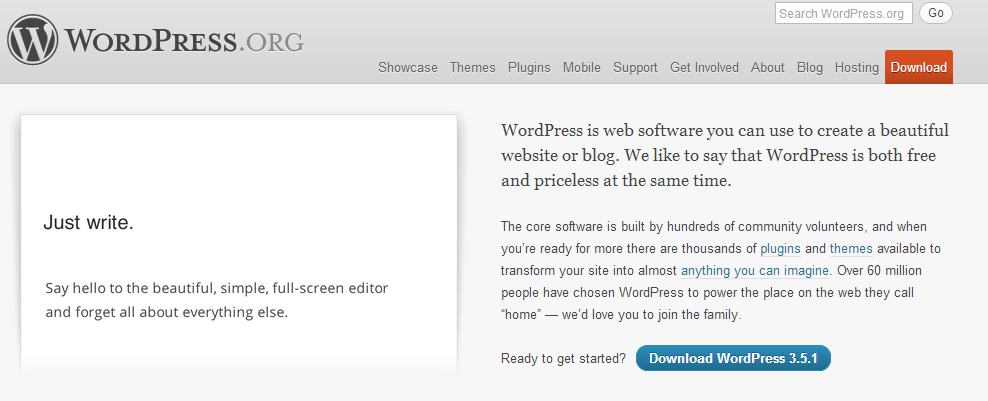The image showcases a web page from WordPress.org, predominantly gray with a darker gray border at the top. This top section features several headers with small words indicating different sections of the website. The WordPress.org logo, represented by a dark blue capital 'W', is prominently displayed.

Dominating the page is a lighter gray background, punctuated by a lighter blue button at the bottom right corner that reads "Download WordPress 3.5.0." Toward the top right, a red header with the text "Download" draws attention.

On the left side, set against a lighter background, are the words "Just Write." Beneath this, a message reads: "Just Write - Say hello to the beautiful, simple, full screen editor and forget all about everything else. WordPress is web software you can use to create a beautiful website or blog. We like to say that WordPress is both free and priceless at the same time." Additional text follows, providing more explanations about the services offered, with highlighted blue keywords like "plugins" and "themes," and a phrase in parentheses: "(anything you can imagine)."

Finally, at the bottom of the page, another call to action appears, highlighted in blue font with white letters: "Download WordPress 3.5.1."